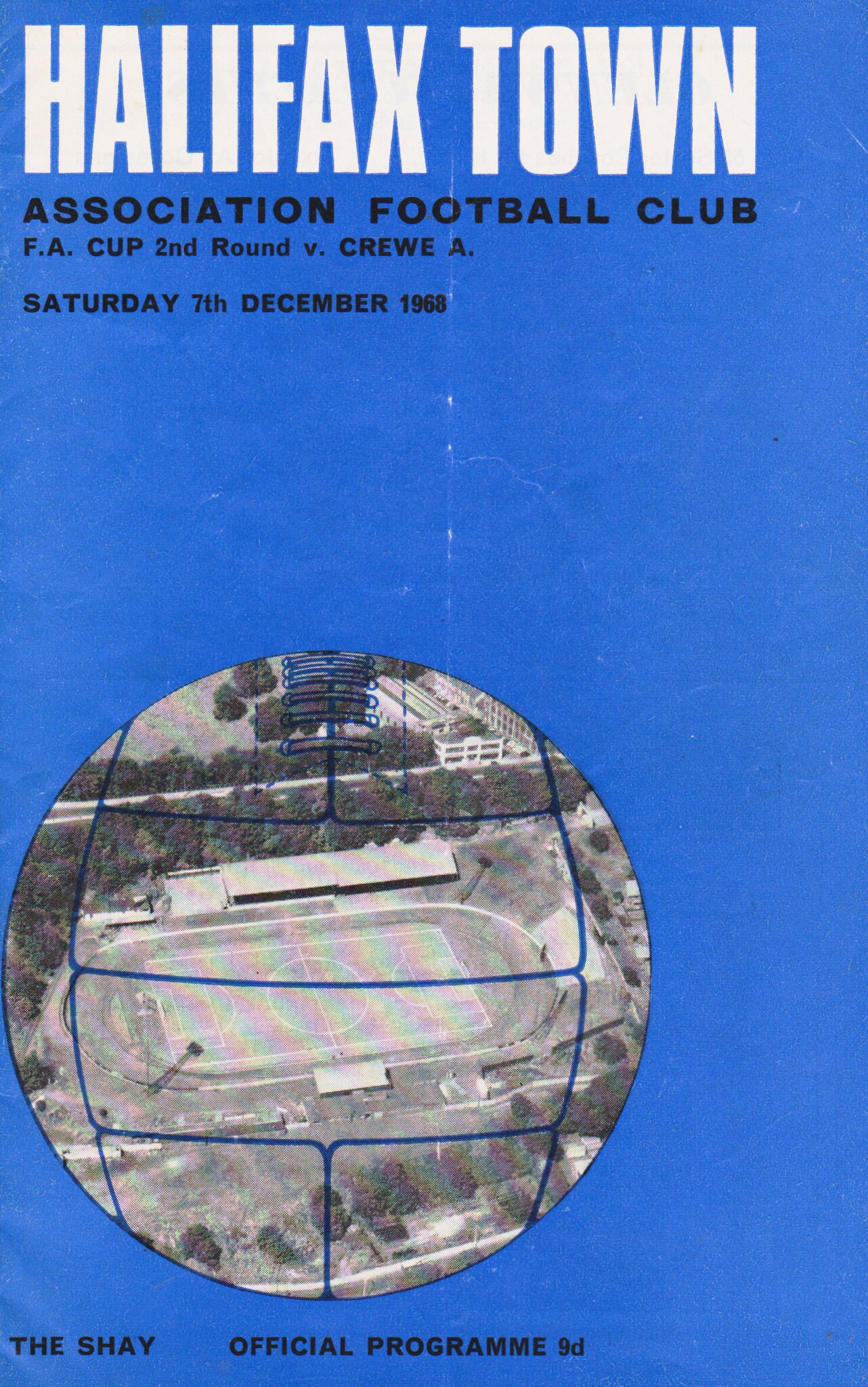The image is of an old, blue soccer program for a sporting event. In bold white capital letters at the top, it reads "HALIFAX TOWN." Beneath that, in smaller black letters, it says "Association Football Club." It lists "F.A. Cup Second Round vs. Crewe A." scheduled for "Saturday, 7th December 1968." The lower portion of the program features a black and white aerial photograph of a soccer stadium, with a blue design drawn within it. Surrounding the stadium are numerous trees. Towards the bottom left, in black capital letters, it says "The Shay," and to the right of that, it reads "Official Program" with the number "9-D" next to it.